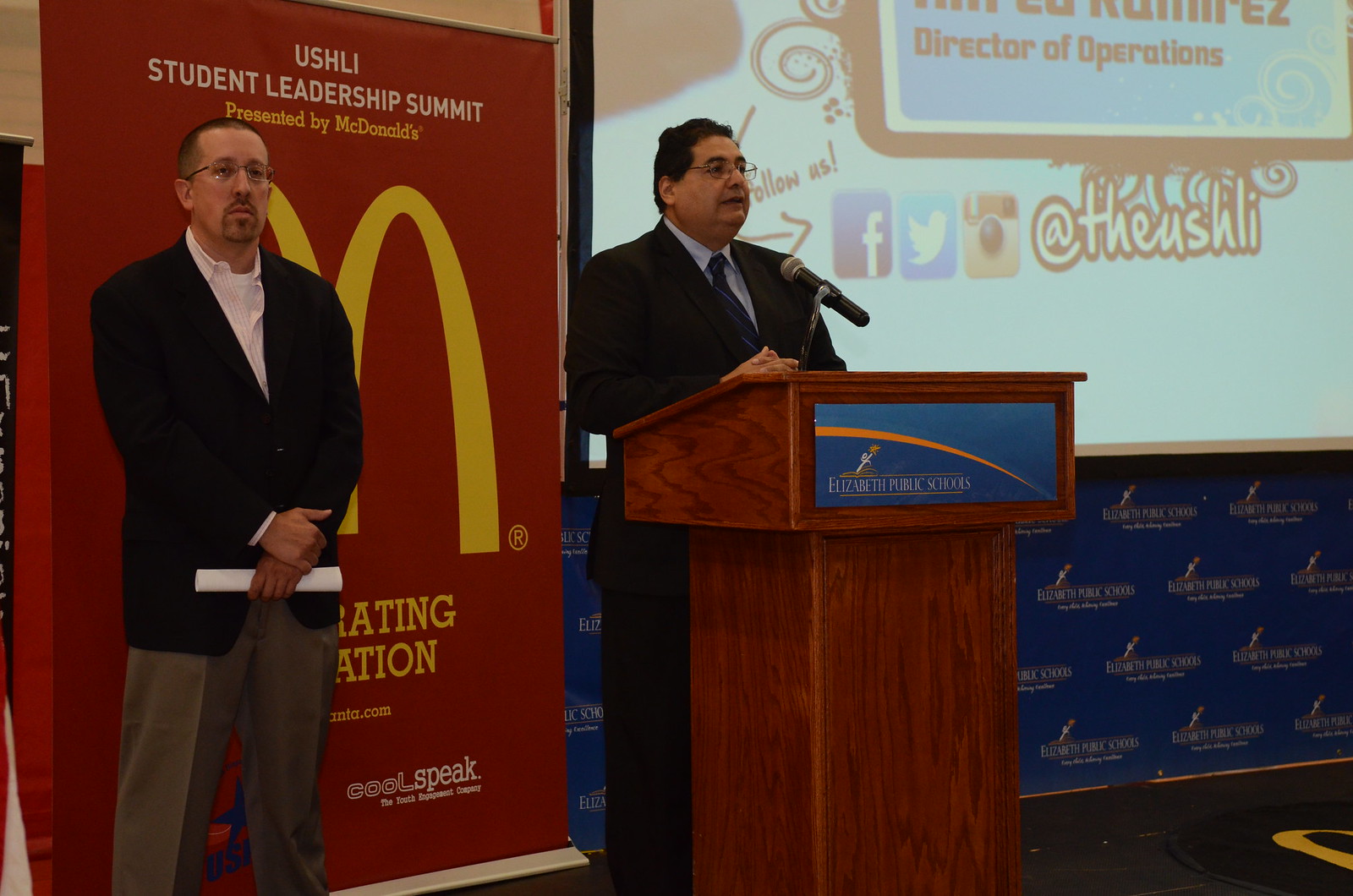The photograph captures a detailed scene inside a building during the UASHLI Student Leadership Summit presented by McDonald's. At the center, an overweight man of light-skinned Hispanic descent, appearing to be in his 40s or 50s, stands behind a wooden podium, passionately speaking into a microphone. He is dressed impeccably in a black suit paired with a blue, white-striped tie and wears glasses. The podium features a blue sign with "Elizabeth Public Services" in white font and an orange arch design. To his left, another man, seemingly in his 30s or 40s and also in a black suit, stands holding a white rolled-up piece of paper. This second man is positioned in front of a large, red banner that prominently displays "UASHLI Student Leadership Summit" in white font at the top and "Presented by McDonald's" in yellow font with the iconic McDonald's 'M'. Additional signage around the podium emphasizes the involvement of Elizabeth Public Schools, reinforcing the event's formal and educational atmosphere.